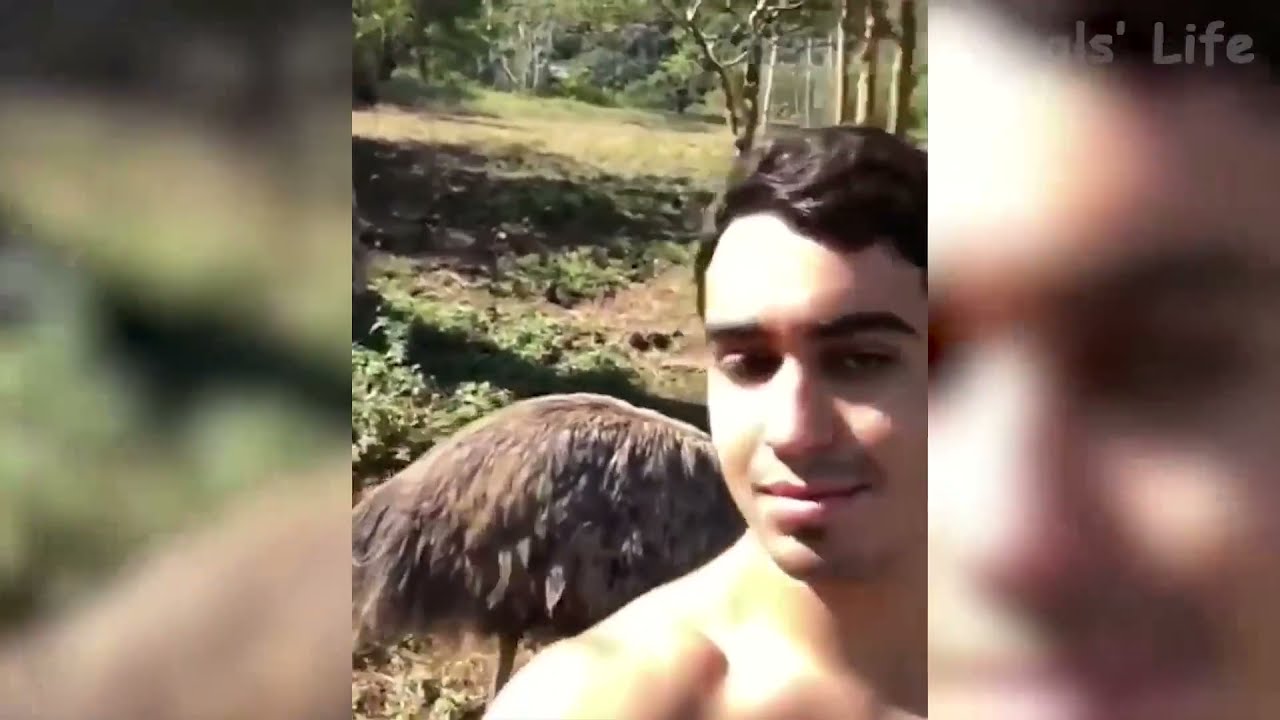A shirtless young man, possibly in his early 20s, with short, dark hair stands very close to the camera, appearing to take a selfie. He has a slight smirk on his face, with closed lips, and is looking directly into the camera. The background reveals a lush, outdoor setting with an extensive grassy area, scattered trees, shrubs, and various plants. Notably, positioned behind him is a large, feathered animal with brown fur or wings that resemble those of an ostrich or emu. The man's head obscures the creature's head, but its slender leg and part of its body are visible. In the top right corner of the image, there is blurred writing that partially reads "life," possibly followed by a name like "Hal's life."